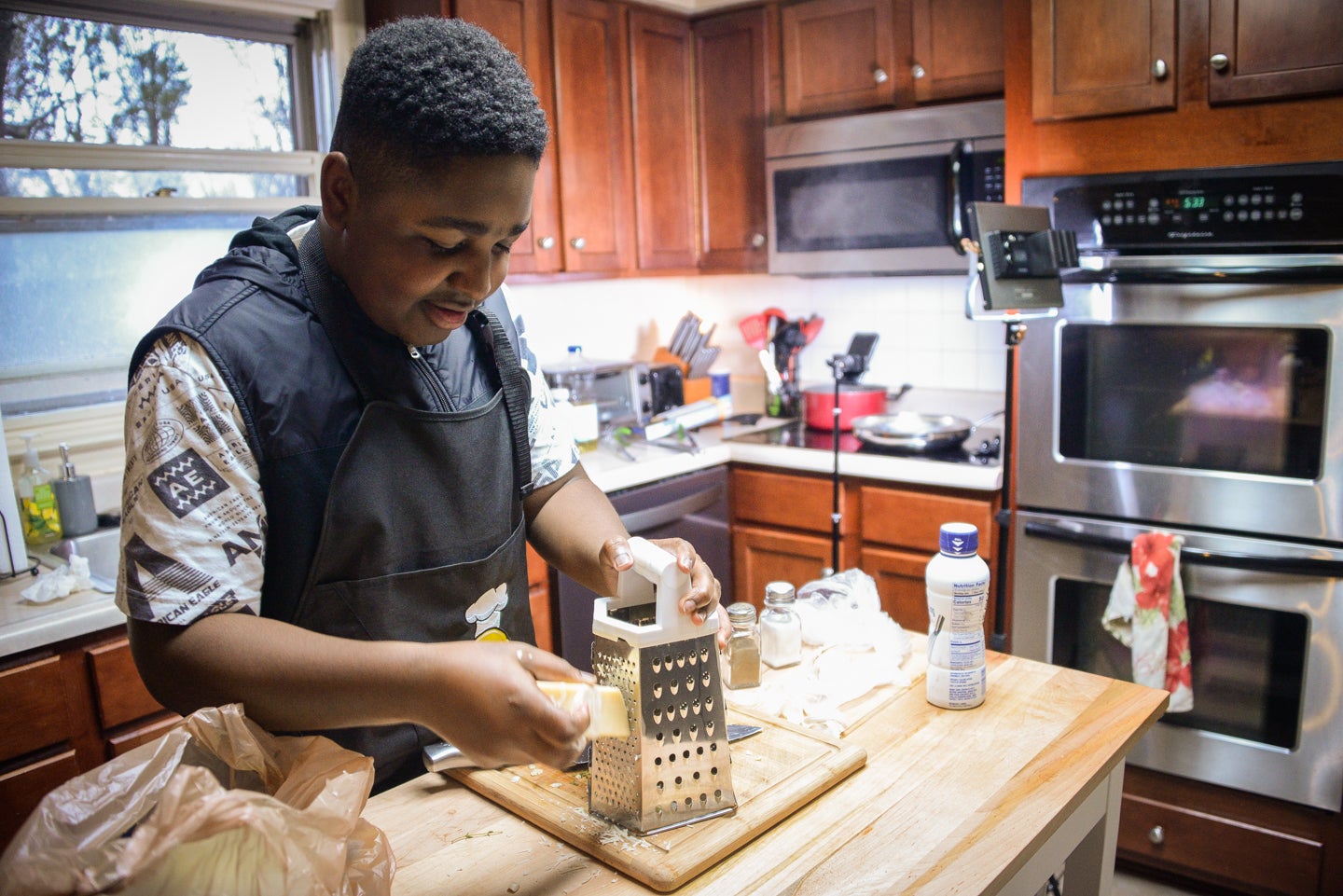In this photograph, a young Black teenager, possibly around 15 or 16 years old, is captured in the midst of preparing food in a bustling kitchen. He has very short, curly hair and is wearing a black chef's apron over short sleeves. Standing behind a central wooden counter, he holds a cheese grater in his left hand and a piece of white cheese in his right, diligently creating shreds on a cutting board. The kitchen around him is busy but organized, filled with various cooking items. A bottle, possibly containing milk or juice, sits nearby on the wooden island. In the background, you can spot a camera setup, hinting that he might be filming a cooking video. The overall ambiance highlights the active and industrious nature of the scene.